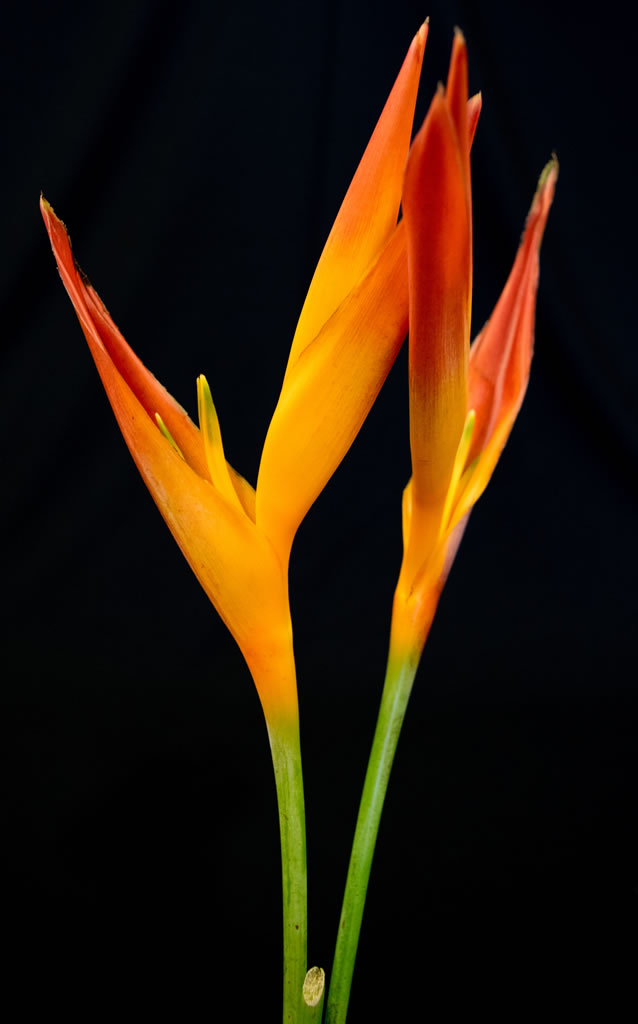A detailed photograph captures two vivid Birds of Paradise flowers against a stark black background. The flowers are mounted on green stems that emerge from a common base, indicating they are part of the same plant. Each flower displays brilliant, gradient colors, with hues transitioning from bright yellow to deep red. Their unique structure bears a striking resemblance to bird beaks, opening widely to reveal vibrant inner parts. Nestled within the flowers are central stems resembling a bird's tongue. The flowers' perpendicular petals encase stamens and smaller inner leaves, adding to their intricate beauty. A third stem at the bottom, cleanly pruned, hints at the plant's previous growth. The black background, devoid of any distractions, accentuates the vivid fluorescence of the flowers, making their health and colors pop vividly.